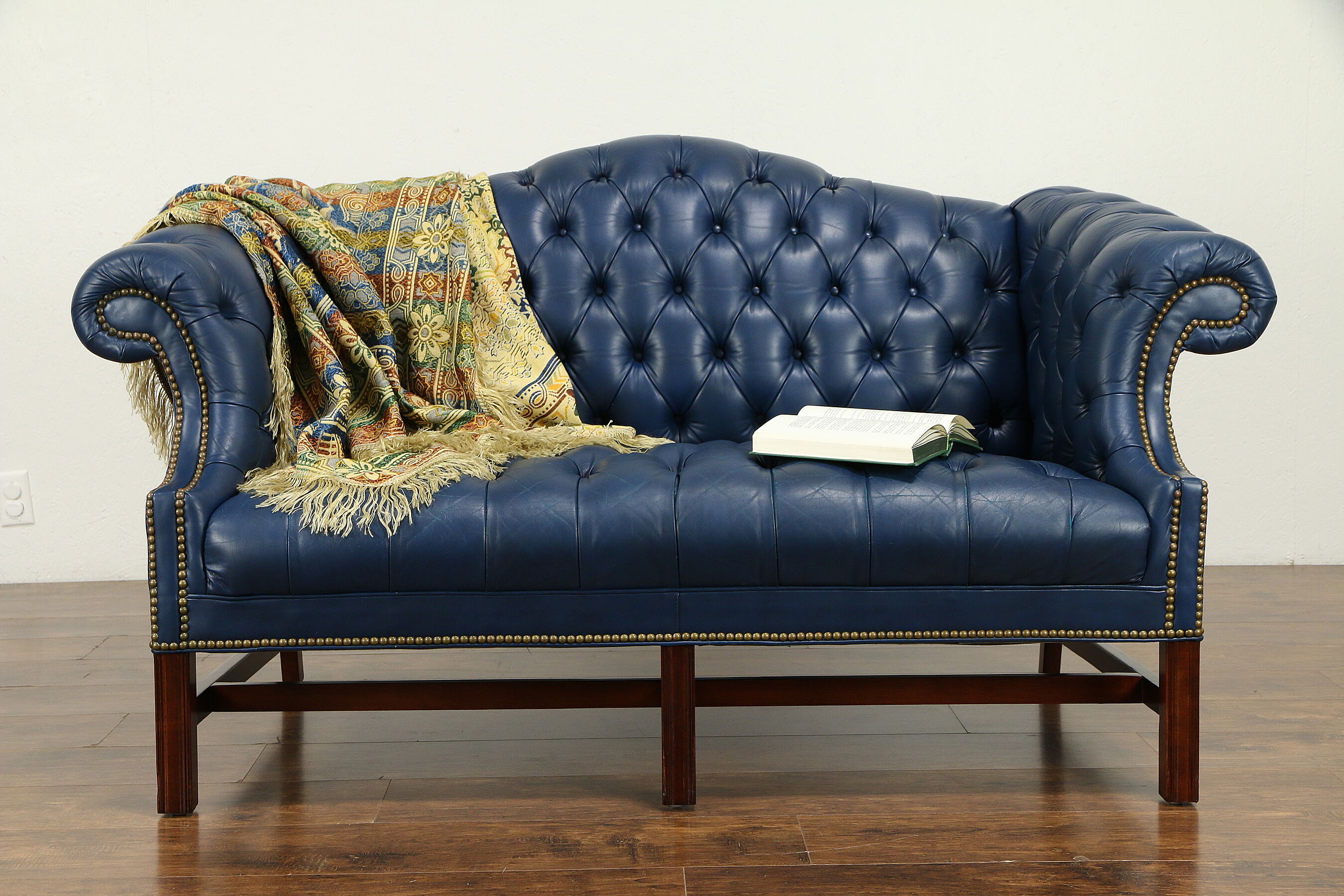This detailed photograph captures an antique, navy blue leather couch with a rich, ornate design, positioned prominently in the room. The couch features a dark brown wooden frame that elevates it slightly above the matching dark brown wooden floor. It is adorned with decorative bronze or gold studs running along the trimming, accentuating its elegance. The back, seat, and sides are intricately gathered to create indented designs adding to its vintage charm. Draped over the left side and back of the couch, there's a luxurious, fringed blanket showcasing a vibrant blend of colors, including gold, blue, orange, maroon, and green, with intricate patterns reminiscent of Indian designs. An open book lies on the right side of the couch, inviting and ready to be read. The backdrop features a white wall with an electrical outlet covered for safety, located towards the left.